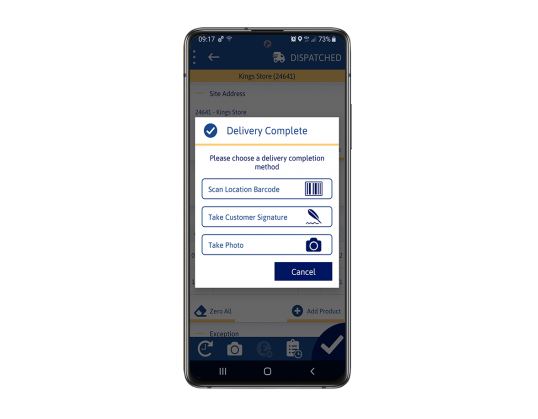The image depicts a cell phone screen displaying various details and options. It is currently 9:17 (the time does not specify if it is AM or PM). The battery is 73% charged. At the top of the screen, there is a back button arrow on the left and the word "Dispatched" on the right. Just below this top row, a yellow bar displays the text "Kings Store 24641" in blue letters.

Beneath the yellow bar, the words "Site Address" appear in blue letters, followed by "24641 Kings Store" also in blue letters. Overlaying the main interface is a pop-up window which is a white rectangle featuring a blue circle at the top, containing a white checkmark and the text "Delivery Complete."

Below the yellow separation bar on the pop-up window, the text reads "Please choose a delivery completion method," with three options listed beneath: "Scan location barcode," "Take customer signature," and "Take a photo." At the bottom of the pop-up, there is a "Cancel" button.

Further down, the cell phone screen shows two additional options at the bottom of the main interface – "Zoom" (or possibly "Zero") on the left side and "Add Product" on the right side.